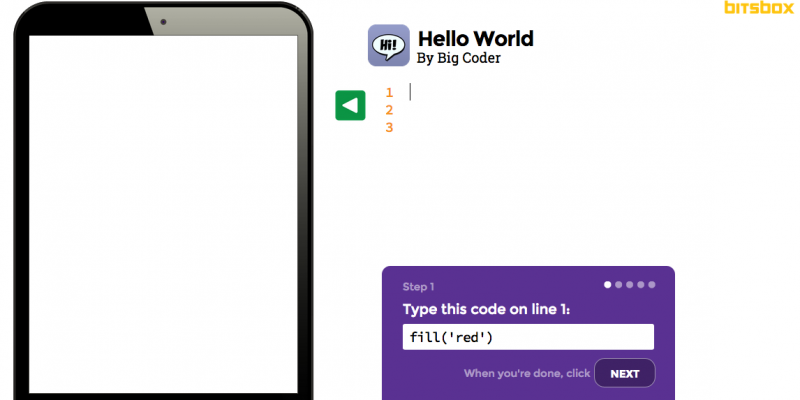To the left side of the image, there is a cell phone. On the right side of the image, starting from the top right corner, the word "BitsBox" appears in yellow lowercase letters with a blocky font style. Below this, center-justified, there is a hot square with a purplish-blue hue containing a speech bubble that says "hi." To the right of this square, the words "hello world" are displayed, followed by the text "bye big corner."

Underneath the speech bubble, there is a play button which resembles a back button. It is a green block with a white triangle tilted to the left, indicating the direction. To the right of this button are the numbers "1, 2, 3." In the bottom right section of the image, there is a purple box labeled "step 1." Below this box, the text instructs to "type this code on line 1."